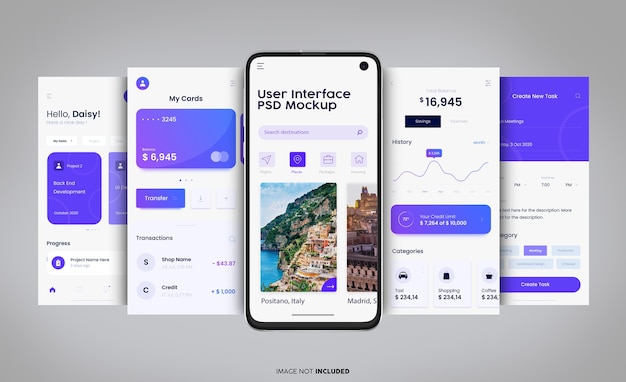This image is a horizontal advertisement for a mobile app, set against a gray background. At the center of the ad is a cell phone with its screen showing a vibrant image of a green mountainside descending to a teal blue ocean, with ruins resembling those found in South American mountain cities. The screen’s purple and white text reads “User Interface PSD Mockup.” On either side of the central phone image are two vertical portrait-oriented screen mockups. 

On the left:
1. A personalized greeting screen with white and purple heading that reads "Hello Daisy."
2. A "My Cards" section displaying an image of a credit card.

On the right:
1. A screen showing a dollar balance and a line chart similar to tracking stock market changes.
2. A "Create New Task" interface.

All the screen mockups use a purple and white color palette with black text. The text at the bottom of the image states, "image dot included."